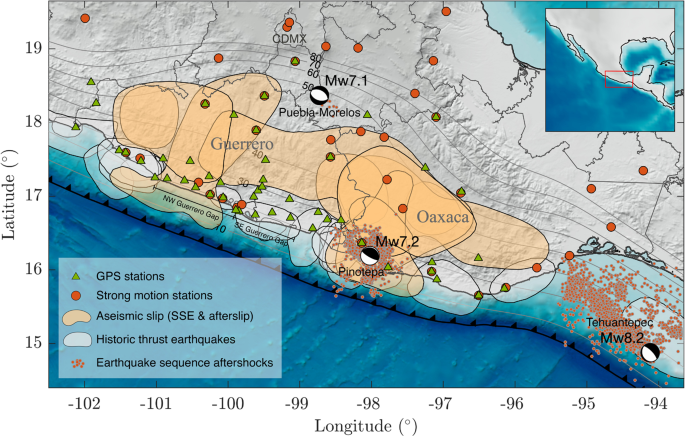The image depicts a detailed map of earthquake activity, likely in Mexico, featuring various geophysical indicators and labeled with specific geographic coordinates. The map spans latitudes from 15 to 19 degrees and longitudes from -102 to -94 degrees. Key locations such as Puebla, Guerrero, Morelos, and Oaxaca are marked, with additional references to Pinotepa. The land area is primarily shaded grey, bordered by a black line representing the coastline, with the ocean to the front.

The map is densely populated with symbols: red dots indicate the earthquake sequence aftershocks, large red circles denote strong motion stations, and green triangles represent GPS stations. Light orange areas signify a seismic slip (SSE and afterslip), while white outlined areas mark historical thrust earthquakes. An extensive distribution of red dots can be seen across the landmass, highlighting regions of intense seismic activity.

In the top left corner, an inset shows an enlarged section of South America with a red box outlining the primary area of interest. The bottom right corner features a comprehensive legend explaining the map's symbols, including green triangles for GPS stations, large red circles for strong motion stations, orange shaded areas for a seismic slip, white areas for historic thrust earthquakes, and conglomerates of red dots for earthquake sequence aftershocks. This detailed and somewhat complex map thoroughly illustrates the seismic characteristics and geographical layout of the area.